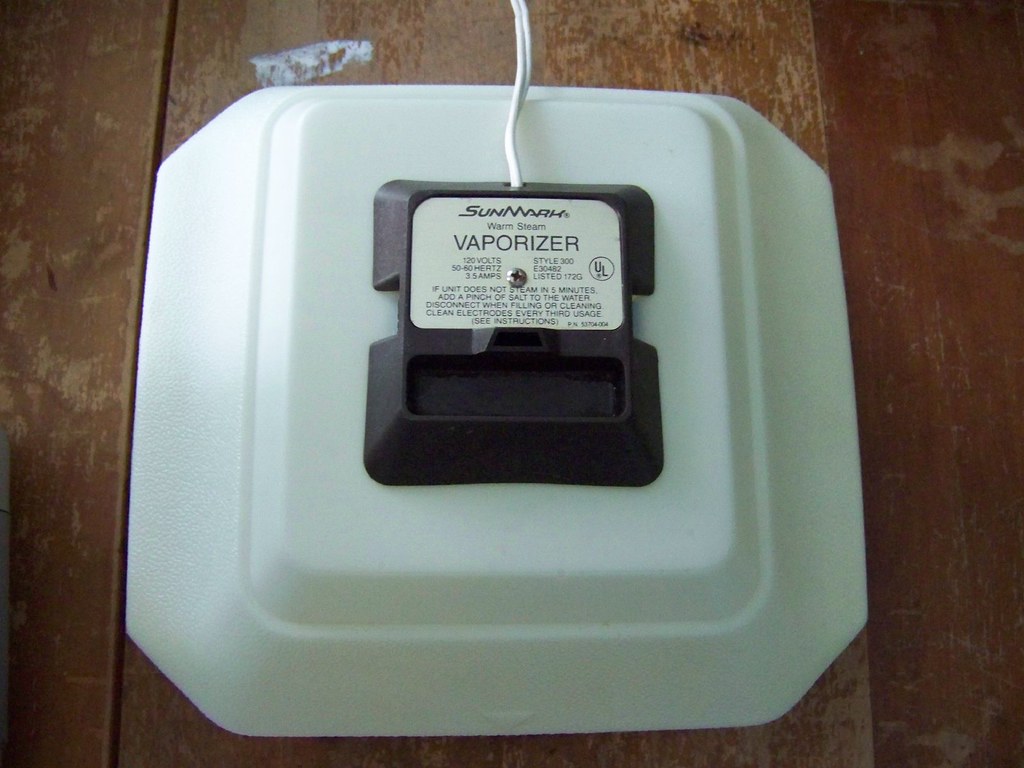This photograph depicts a white Sunmark Warm Steam Vaporizer prominently placed in the center of the image, resting on what appears to be a brown wooden floor, characterized by visible slats and signs of discoloration. The vaporizer features a black back panel, which includes detailed labeling of the brand and operational instructions. A white cord extends from the vaporizer, indicative of the power connection. The image is a close-up, focusing exclusively on the vaporizer, with no other items or text visible in the frame. The colors in the image are predominantly white, black, and brown, harmonizing with the wooden floor backdrop.